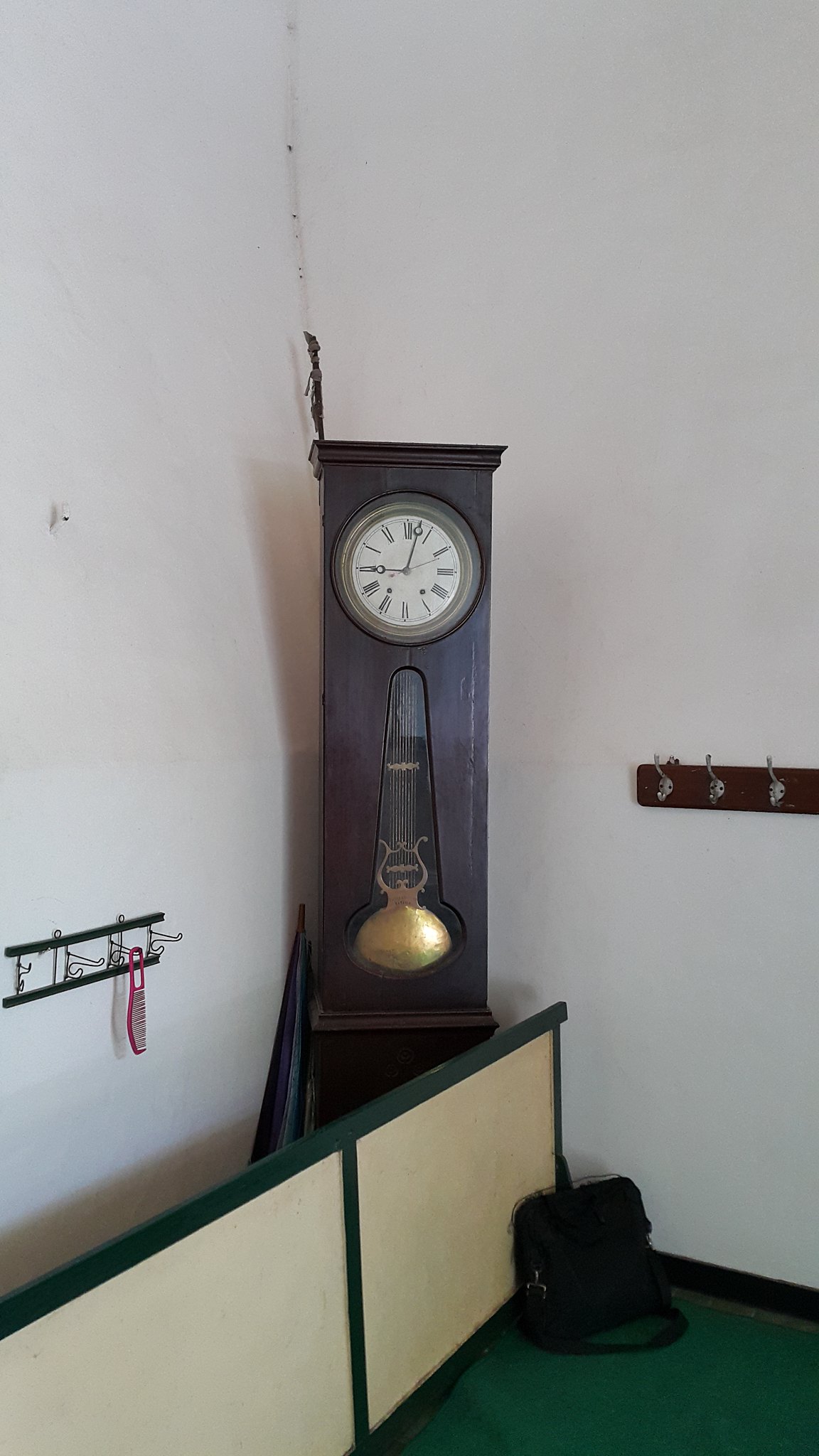This photograph captures a cozy corner of a room with white walls and a green carpeted floor. Dominating the scene is a small, upright grandfather clock made of dark cherry wood, situated precisely at the room's corner. Its round, white face with Roman numerals shows the time as just past nine o'clock, with the minute hand at twelve, the hour hand at nine, and the seconds hand slightly past the ten. Below the clock face, the brass pendulum is visible, swaying within its wooden casing.

To the right of the grandfather clock, mounted on the wall, is a brown rectangular wooden piece with three silver hooks, intended for hanging coats. To the left of the clock, there is a green rectangular metal frame, about knee-high, with a pink hairbrush with white bristles hanging from it. Leaning against the clock is a dark and light blue striped umbrella. On the floor in front of the clock, partially obscuring its base, is a green rectangular area rug adorned with beige squares, bordered by green lines. This rug extends towards the lower left corner of the photograph.

In addition, a black bag with a strap is situated near the wall, appearing to be leaning against the knee-high green metal frame. The room’s arrangement includes these various items, creating a sense of lived-in comfort and practical organization.